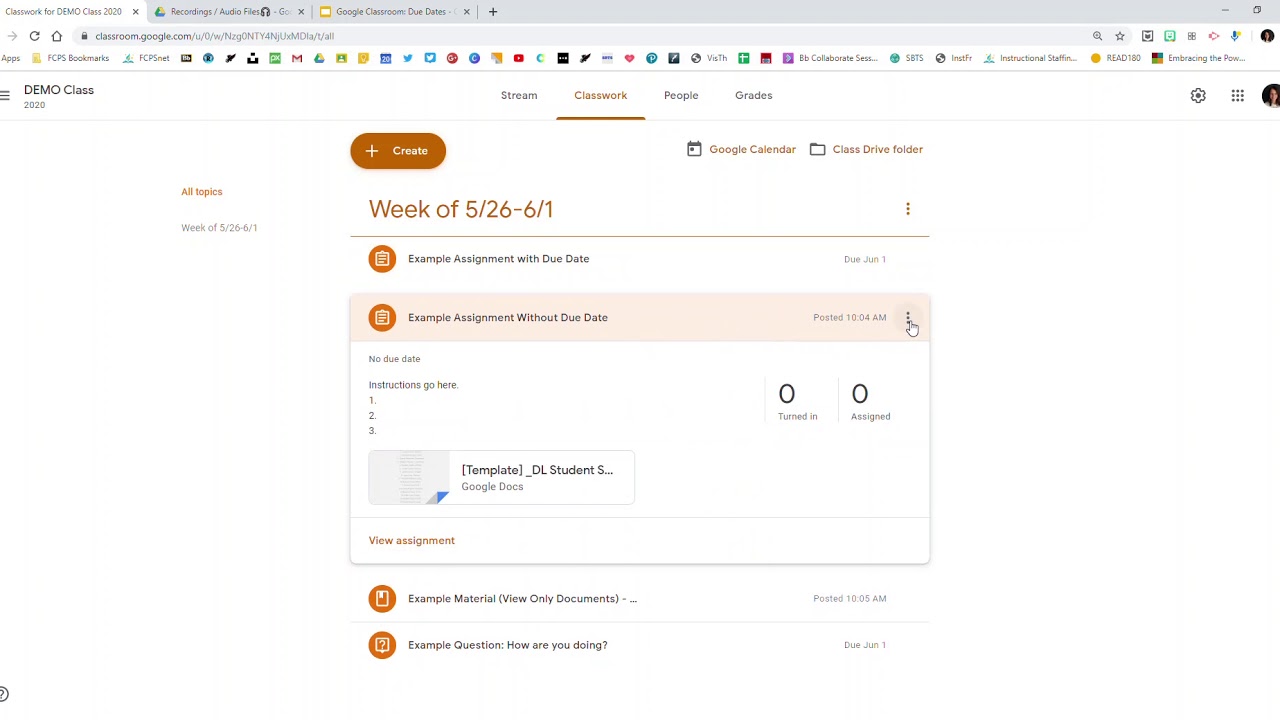A detailed teacher's lesson plan for a virtual class is showcased on a Google Classroom interface. In the top-left corner, a header reads "Classwork for Demo Class 2020." Adjacent tabs include "Recording/Audio Files" and "Google Classroom Due Dates." The browser's address bar displays the URL "classroom.google.com," followed by a string of alphanumeric characters.

The left sidebar features menu options: "Demo Class 2020," "Stream," and underlined "Classwork," along with "People" and "Grades." An orange box prominently displays a plus sign and the word "Create" in white text. Icons of a calendar and a folder are labeled "Google Calendar" and "Class Drive Folder," respectively.

The instructional content is organized by the week of 5/26 to 6/1. Listed assignments include "Example Assignment with Due Date - due June 1" and "Example Assignment without Due Date - posted at 10:04 AM, No Due Date." These assignments are followed by placeholder instructions indicated by numbers 1, 2, and 3. An attachment named "Template_DL Student Google Docs" is available, followed by a link to "View Assignment."

Further down, it lists "Example Material - View Only Documents" and an example question asking, "How are you doing?" with a due date of June 1.